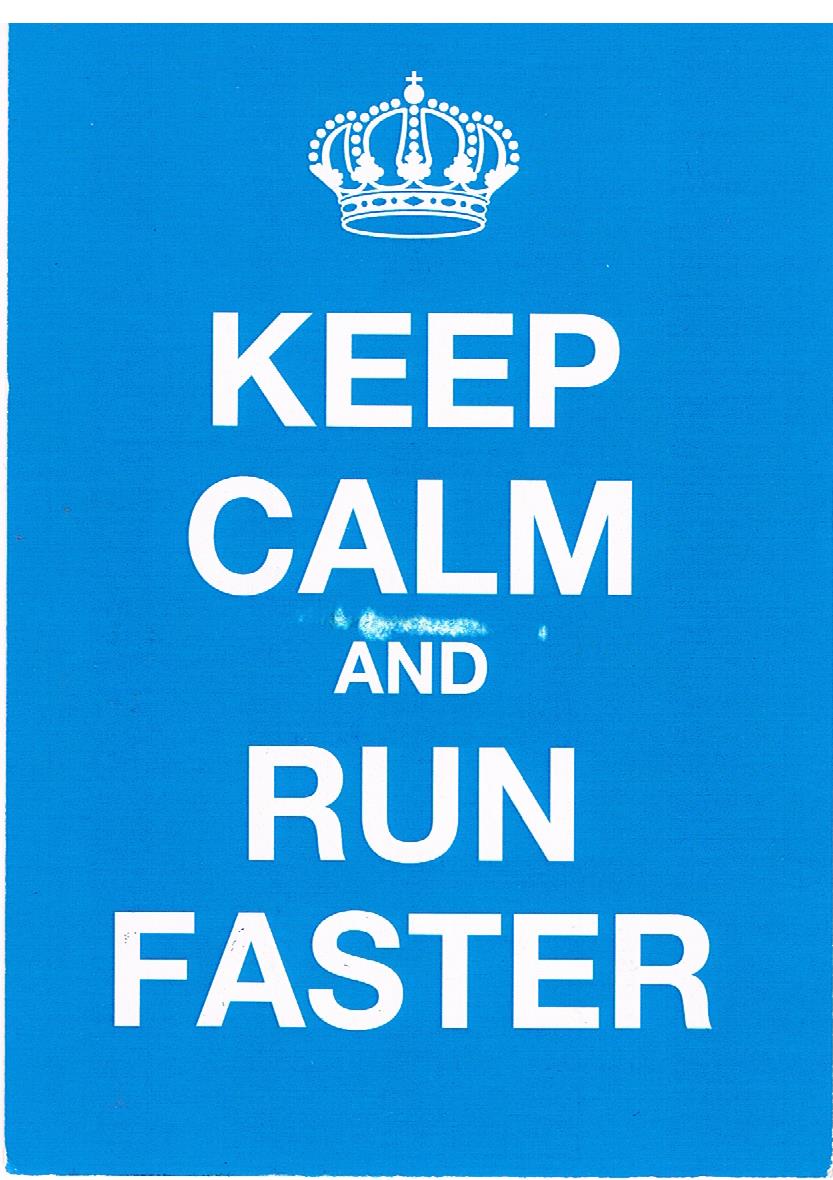This rectangular digital poster features an inspirational message, prominently displayed on a blue background. At the top, a detailed white drawing of a bejeweled crown with a small cross at its peak captures the viewer's attention. Directly beneath the crown, in bold, all-capital white letters, the motivational text reads "KEEP CALM AND RUN FASTER." This message is structured across five separate lines, with varying font sizes: "KEEP" and "RUN FASTER" are notably larger, while "CALM" and the connecting "AND" appear smaller. Subtle imperfections add a touch of authenticity to the design—there are visible signs of wear above the "AND," and faded white patches suggesting wear and tear, particularly around the middle and bottom corners.